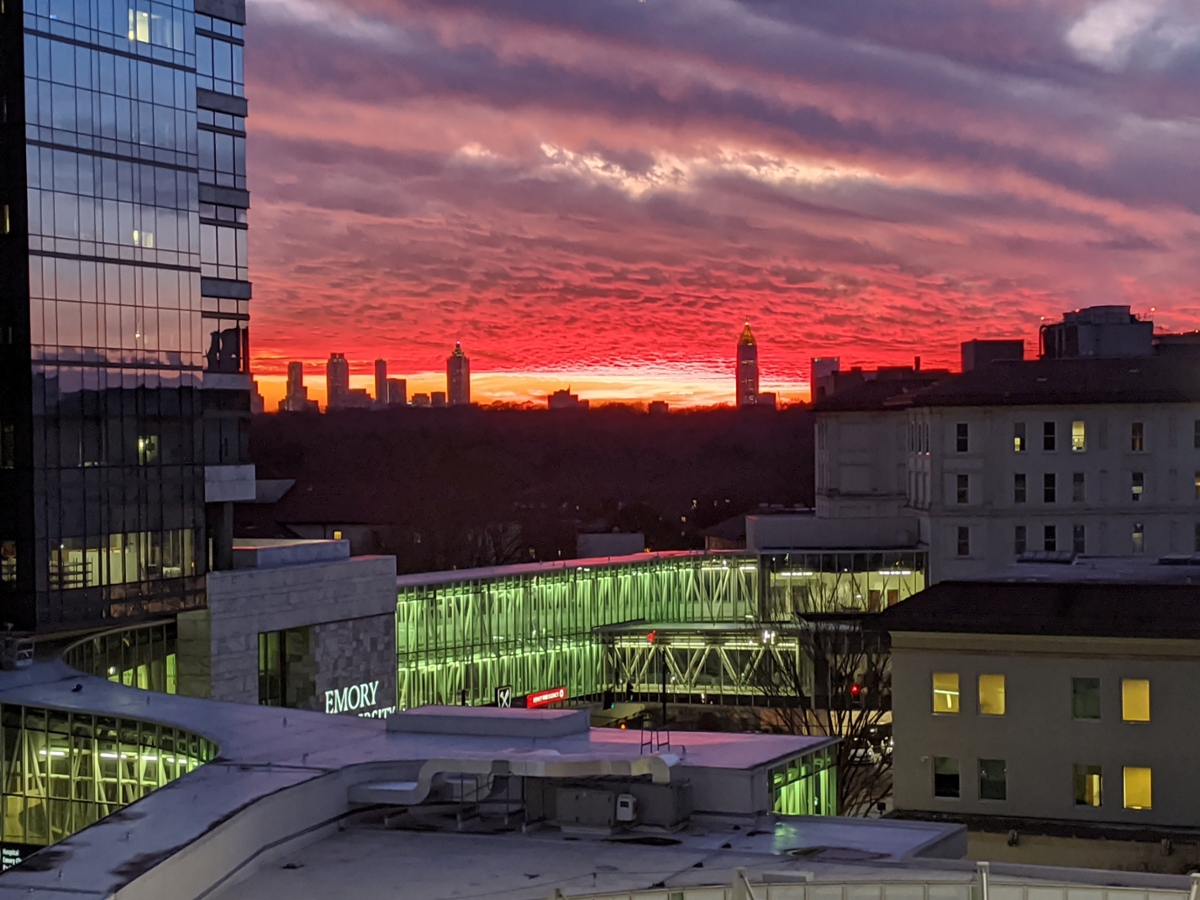The image captures a vibrant city scene at sundown, where the sky transitions dramatically from bright orange to a soft pink, and finally to a deep purple. Central to the scene is a large skyscraper on the left, towering with glass windows framed in black. Adjacent to this prominent structure is another tall building, both of which dominate the skyline alongside smaller buildings. Two distinct sections can be seen at the bottom half of the image; the front of a building with light green windows illuminated, supported by white structural bars, creating a sense of division. Amongst the cityscape, there is a building labeled "Emery," featuring a glass-walled walkway designed for panoramic views. The right side of the scene displays smaller buildings with white walls and dark gray roofs. The urban environment is further enriched by a leafless tree, adding a stark, natural contrast to the architectural forms. Clouds densely populate the sky, allowing minimal glimpses of the sunlight casting a warm glow over the city.